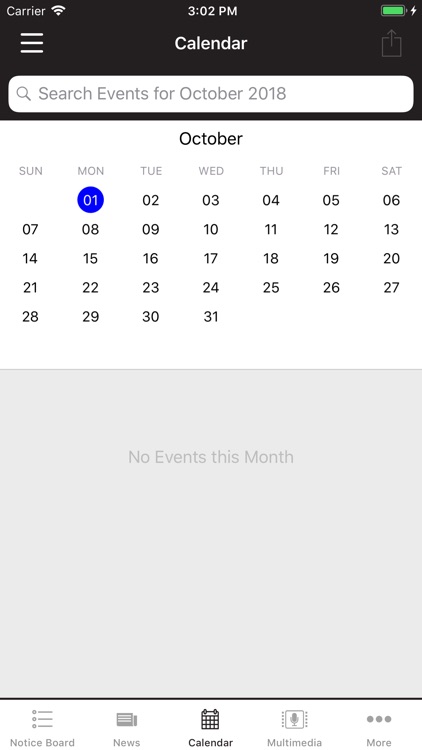**Caption:**

The image shows a detailed screenshot of a phone’s calendar interface from October 2018. At the top, the status bar includes the carrier information on the top left, a Wi-Fi icon, the time "3:02 PM" centered, and a green battery meter with a lightning bolt indicating it is currently charging on the top right. Below the time, "Calendar" is displayed in white text on a black horizontal bar, which is part of the background color.

On the left side, beneath the carrier information, three horizontal lines are visible, which likely serve as the menu icon. Below these lines is a search bar for finding events. The calendar view shows October 1st highlighted with a blue circle, marking a Monday. Underneath the date, a box states "No events this month," written in light gray text.

Further down, the interface includes five different icons: a notice board, news (greyed out), a calendar, a multimedia button, and three dots for more options. Directly below these icons, a share button is present, allowing users to share the calendar. The primary colors in the screenshot are white for the calendar background, black for text, light gray for notice areas, blue for the selected date, and green for the battery meter.